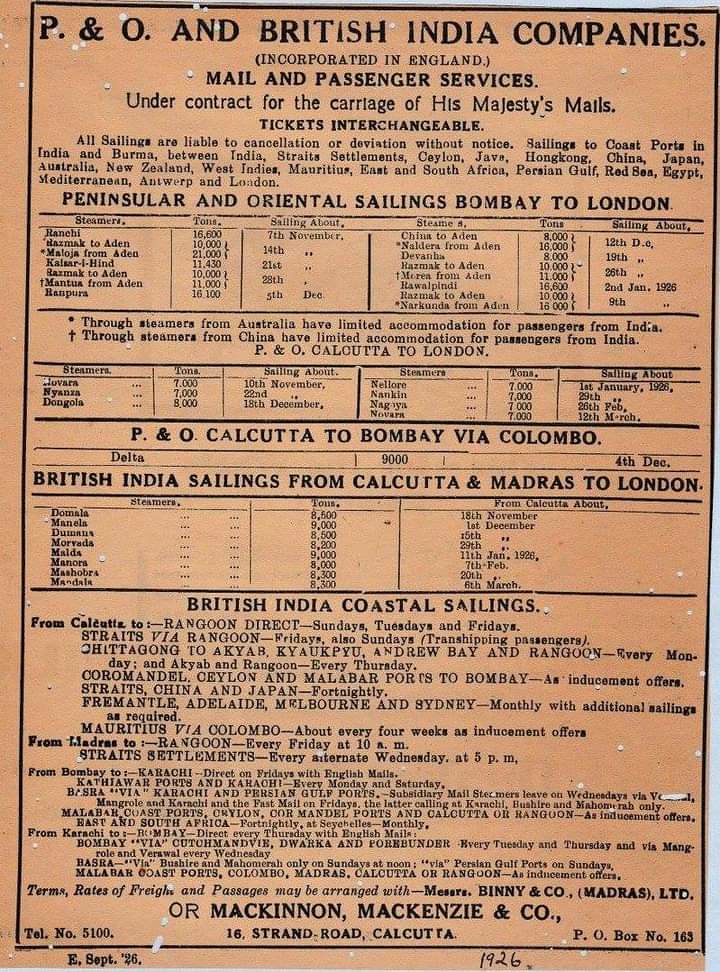This image is a vintage printed publication that serves as a schedule for mail and passenger services operated by the P&O and British India Companies. The entire image is dominated by text, primarily in black, set against an aged, tan or yellowish parchment background that hints at its vintage nature. The headline at the top reads: "P&O and British India Companies Incorporated in England," followed by details about their mail and passenger services under contract for the carriage of His Majesty's mails, with the note that tickets are interchangeable and all sailings are subject to cancellation or deviation without notice.

Various schedules and routes are specified in a series of subheadings and columns. First, the "Peninsular and Oriental Sailings" cover routes from Bombay to London. Below this, the schedule for "P&O Calcutta to Bombay via Colombo" is listed, followed by "British India Sailings from Calcutta and Madras to London." Additional schedules detail "British India Coastal Sailings," with specific routes from Calcutta, Madras, and between Bombay and Karachi. The extensive list of ports includes India, Burma, Straits Settlements, Ceylon, Java, Hong Kong, China, Japan, Australia, New Zealand, West Indies, Mauritius, East and South Africa, Persian Gulf, Red Sea, Egypt, and the Mediterranean.

At the bottom, it mentions that terms, rates of freight, and passage may be arranged with "Monsieur's Binion Company, Madras Limited," or "McKinnon McKenzie and Company" with their address at 18 Strand Road, Calcutta. The date "1926" is handwritten at the bottom edge, further anchoring it in its historical context. Overall, the piece is a comprehensive and intricately detailed advertisement or schedule reflective of early 20th-century travel logistics.